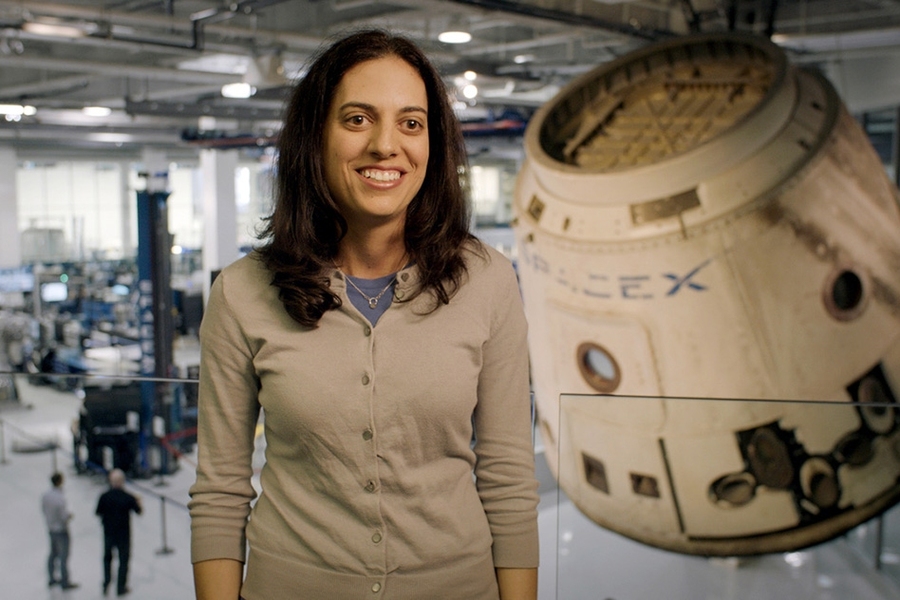In the image, a woman is the central focus, standing and smiling warmly, showcasing her brownish-black shoulder-length hair with a slight wave. She is dressed in a somewhat unattractive beige-green button-up shirt with a blue undershirt. The woman, possibly in her 30s, has large hazel eyes and tan or brownish skin. Around her neck, she wears a gold ring necklace, adding a subtle touch of elegance.

The background features the bustling environment of the SpaceX factory floor, which is somewhat blurred, but still reveals key details. The area is characterized by its industrial atmosphere, complete with heavy lifting equipment such as forklifts and CNC machines, assembly lines, and extensive HVAC installations on the ceiling. In the bottom left-hand corner, two men are seen conversing; one is dressed in black and the other is wearing a grey shirt.

Prominently to the right of the lady hangs a significant focal point: a large, white SpaceX capsule suspended from the ceiling. This capsule bears the blue SpaceX logo and shows burn marks from atmospheric re-entry, underscoring its monumental journey through space. Despite the blur, the overall scene suggests a dynamic setting likely within a space center or space museum, evidenced by certain elements like roped-off areas and informational screens traditionally seen in such environments.